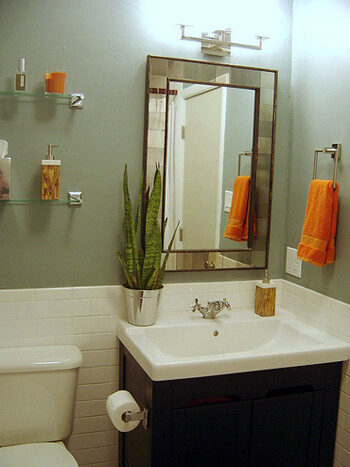This photograph captures a stylish and minimalistic bathroom interior. The focal point is an elegant mirror above the sink, framed by small square mirrors that add a touch of glamour. Hanging to the right of the mirror is an orange hand towel, adding a pop of color to the space. Below the mirror, there is a soap dispenser and a small potted plant, which appears to be artificial, enhancing the sink's decor.

The sink itself is a standard white basin with a wooden tan cabinet beneath it, offering some storage. Attached to the left side of the cabinet is a toilet paper holder, and just to the left of that, you get a partial view of the toilet. Above the toilet, several small shelves are mounted on the wall, holding various items such as lotion, tissues, a toothbrush holder, and possibly some nail polish or makeup.

The bathroom’s design is crisp and clean, featuring a light gray paint on the upper walls and white tiles on the lower half. The overall aesthetic is minimalist yet functional. Illuminating the space, two light sconces are mounted above the mirror, providing ample light for the vanity area.